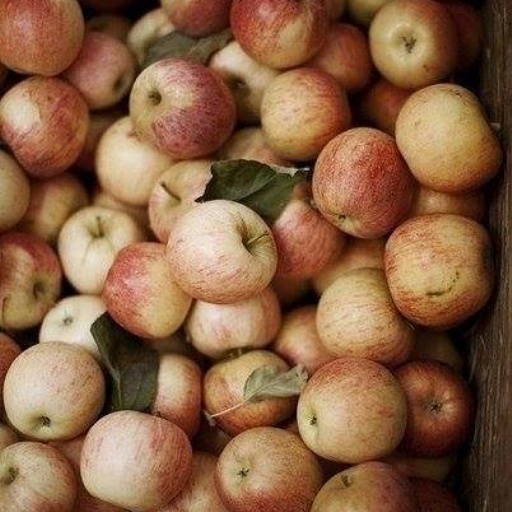The image showcases a large pile of red and yellow apples, each with green stems. Some apples still have small green leaves attached, which appear a bit crumpled, indicating they may have been recently picked. The apples are interspersed with one another, creating a vibrant mix of red and yellow hues. A few apples display small black spots, with one spot resembling a bite mark. The apples rest against a visible wooden wall to the right, and it's unclear if they are on a wooden table or the ground. The scene suggests an abundant harvest, with over 50 to 60 apples stacked together, looking fresh, delicious, and juicy.